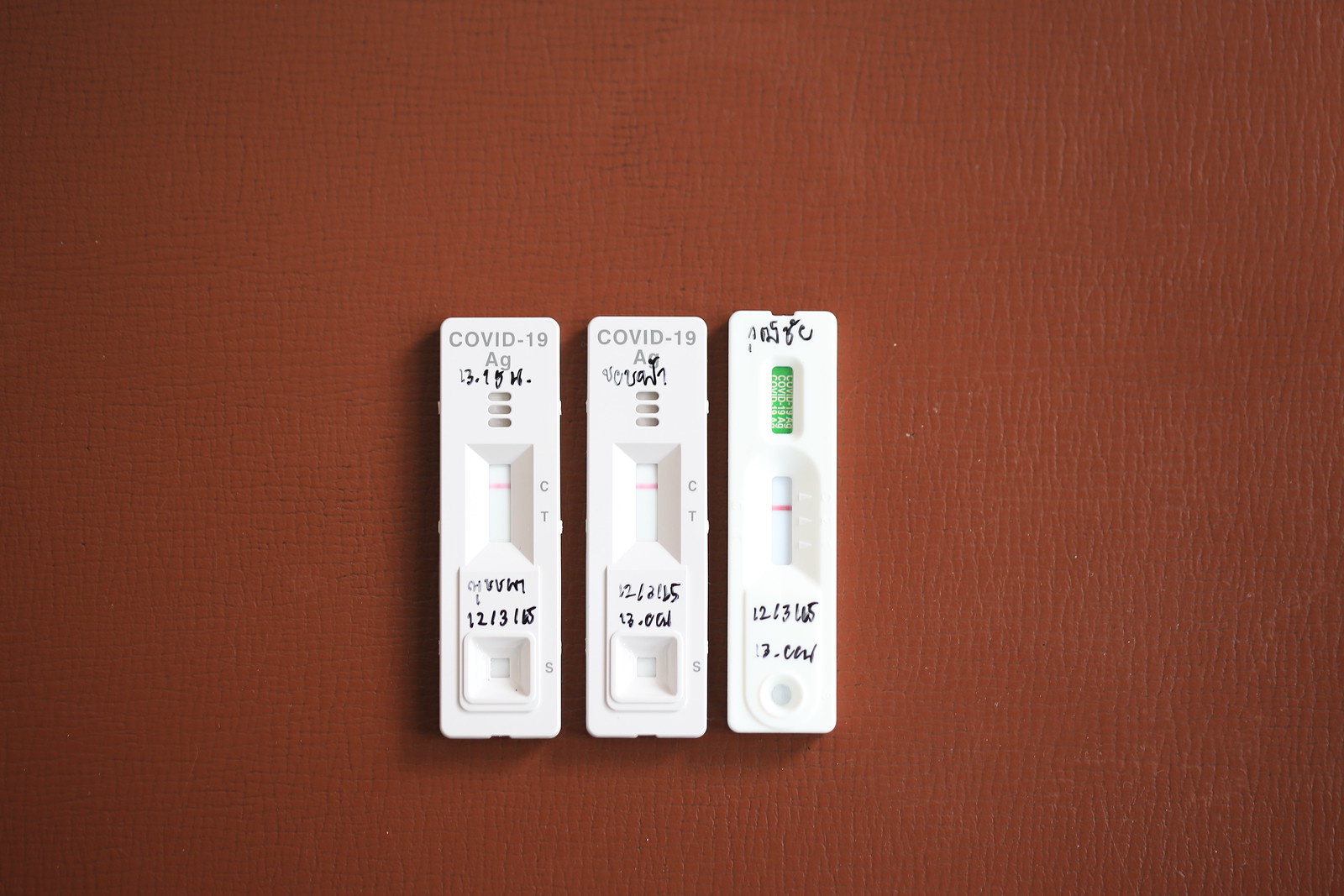This horizontal, rectangular image showcases three small, vertical test devices at its center, set against a rustic brown, vinyl-like background. The tests are all made of white plastic. The first two devices are marked with "COVID-19" in light gray text, followed by "Ag" in smaller letters. These two tests are identical, each featuring three vertically aligned, indented fields at the top. Beneath these fields, there is a sunken rectangular window labeled with a "C" and "T" on the right side. A horizontal red line appears at the "C" position on both tests. Additionally, black marker inscriptions are visible under the "Ag" on these tests, and there is another sunken square area marked with an "S".

The third test differs from the first two. It has illegible text written in black marker at the top. A small vertical inset area highlighted in green with white lines is located beneath the marker text. Like the other tests, it has a sunken rectangular window with a horizontal red line and some black writing. At the bottom, a sunken circular area is visible. The overall composition and details of these test devices are clearly depicted against the textured brown background, providing a vivid and descriptive visual reference.